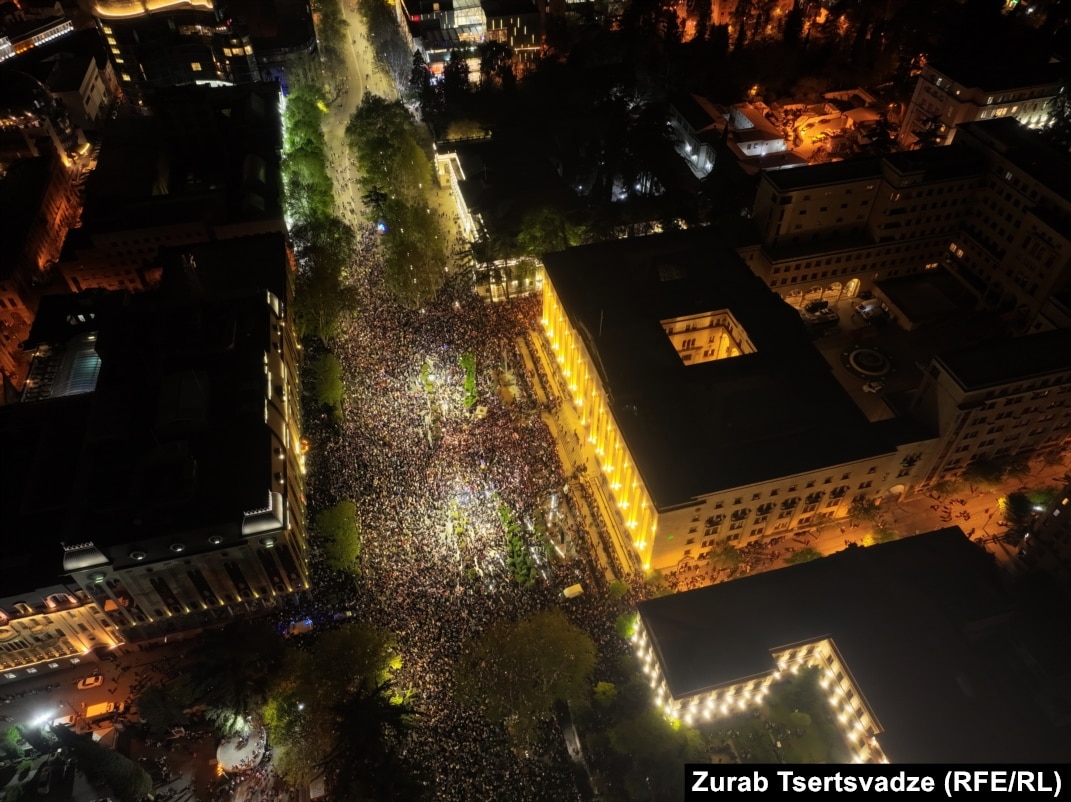This aerial nighttime photograph, likely taken from a drone or helicopter, captures a dramatic scene in a city. The street, lit dimly by the buildings on either side, runs from the bottom middle of the image and veers slightly to the left, continuing out of frame just off-center at the top. The street is teeming with thousands of people, who are swarming around stopped cars. The crowd is most densely packed between two prominent buildings—a large one just right of center with a distinctive rectangular hole in its roof and another across from it. Both buildings, like others in the image, are four to five stories tall and emit a yellowish glow that illuminates the scene. The rooftops appear black, adding to the dark ambiance. The street is lined with trees, and their canopies are visible above the throng. The presence of people diminishes slightly as one looks further up the street, but the lower section remains densely crowded. In the bottom right-hand corner of the image, there is a watermark with the name "Zurab Tsertsvadze (RFE/RL)" in white text.